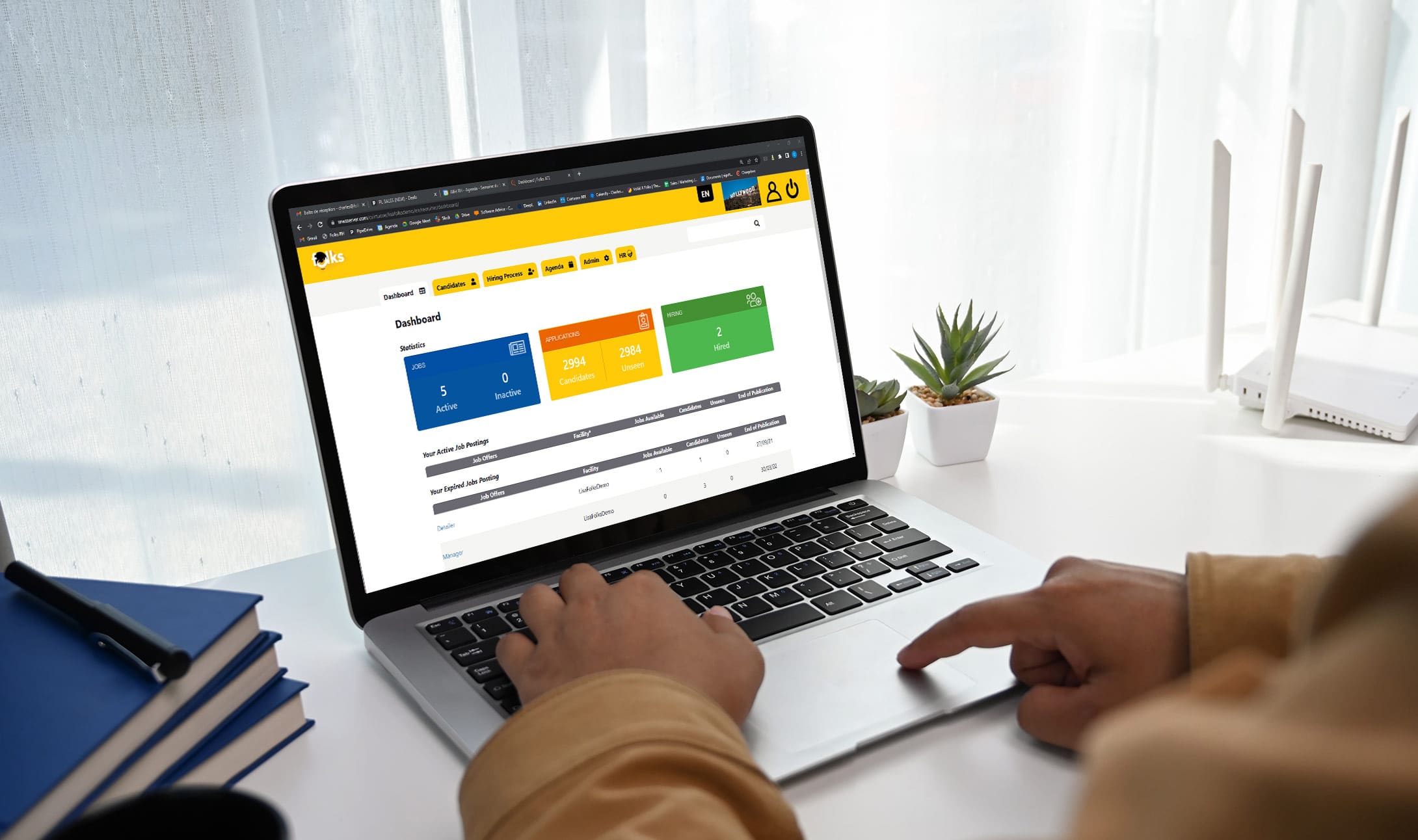A person with dark skin, dressed in a brown long-sleeve jacket, is seated at a white desk that stretches across the entire width of the photo. The individual is engaged with a laptop, their left hand poised on the keyboard and their right finger on the trackpad. The laptop screen displays three prominent rectangles in blue, red and yellow, and green.

In the foreground, on the left side of the desk, three blue books are stacked unevenly, each one slightly askew from the one below. A black strap or handle is draped across these books, adding a casual detail to the arrangement. Partially visible in the corner is a coffee cup.

Behind the desk are windows, evidently dirty and needing cleaning. They appear foggy with droplets of moisture trickling down, suggesting a cold interior and a warmer exterior environment.

To the right of the laptop, two small white planters hold green succulents, adding a touch of nature to the workspace. Further along the desk, an object that resembles an upside-down piece of tech equipment with visible legs is situated, contributing to the workspace's eclectic feel.